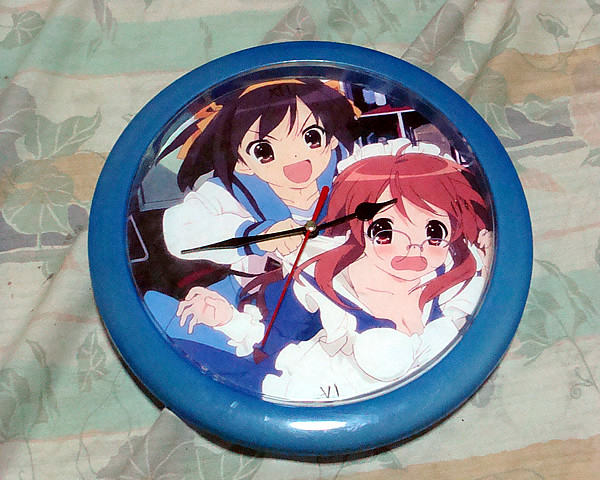The image portrays a detailed, multi-layered scene. The background consists of several photographs arranged in a gradient from top to bottom: light at the top, followed by green, then white, and brown at the very bottom. To the far right, the colors white and brown are also prominent.

At the center of the image is a clock encased in a ceramic-like, blue plastic material. The clock face features second hands pointing downward to the left, and a smaller hand pointing directly to the left.

Superimposed on the clock is an anime illustration featuring a character who appears to be Hiroki Muzio, positioned at the top of the image. She has an orange band and is depicted pulling on another character in front of her. The character being pulled wears glasses, has red hair, and is adorned in a white frill and apron over a blue blouse with white sleeves.